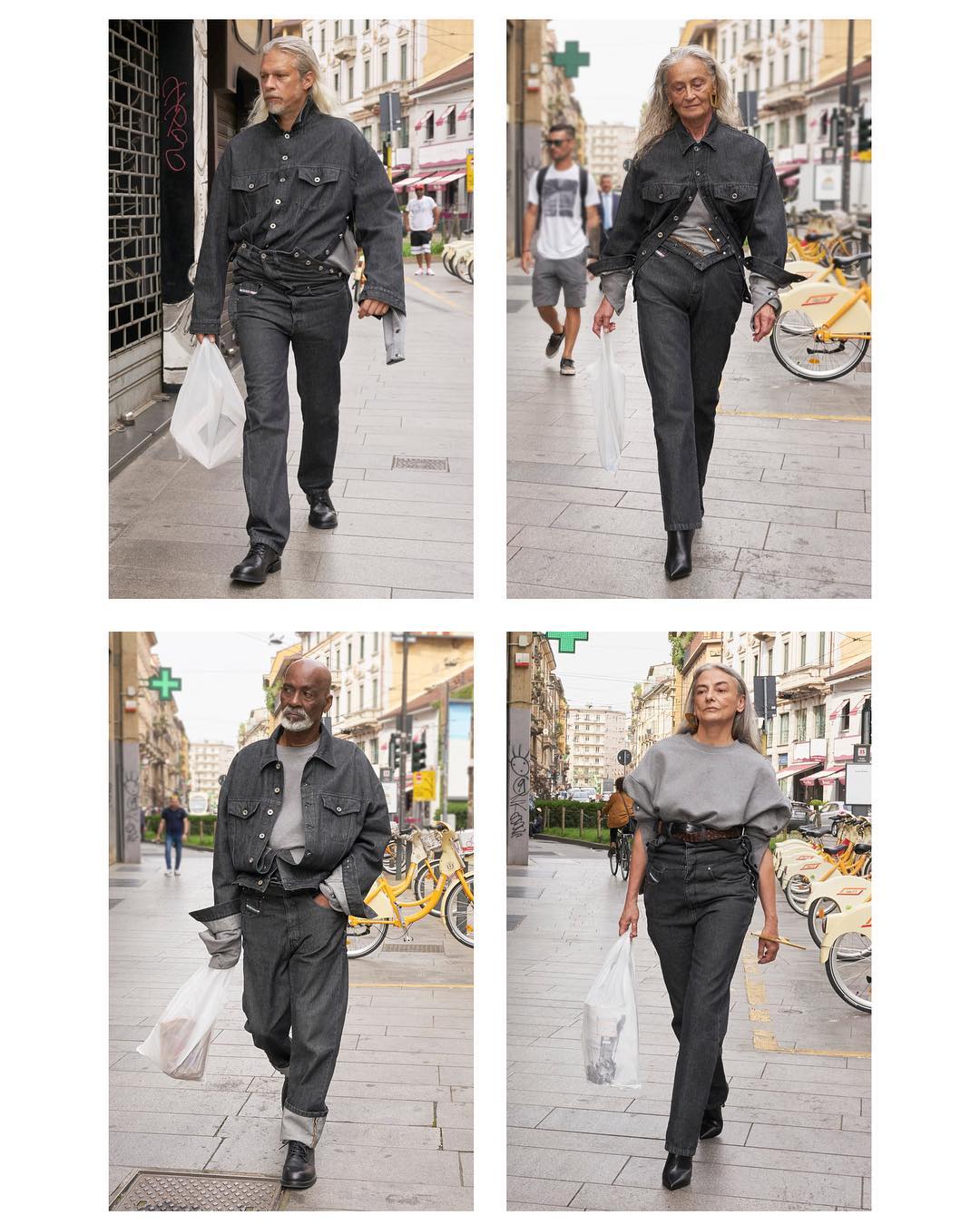The image is a collage featuring four vertical rectangular photos, each depicting a different elderly individual dressed similarly, with slight variations in their outfits. The top left photo shows a man with long gray hair and a goatee, wearing black jeans, a black denim button-down shirt partially tucked into his pants, and black leather shoes; he's carrying a white grocery bag in his left hand. The top right photo is of an elderly woman with long gray hair. She is dressed in black jeans and a black denim shirt with only the top two buttons fastened, revealing a gray shirt underneath. A street scene with a man, a backpack, sunglasses, and bicycles is visible behind her. The bottom right photo features another elderly woman with long gray hair. She is dressed in black jeans, a gray sweater instead of a denim shirt, black shoes, and is also holding a white grocery bag. Bicycles and a cobbled street are visible in the background. The bottom left photo shows an older black man with a beard and a bald head. He wears black jeans, a black denim button-down shirt with the sleeves rolled up once, a gray shirt underneath, and black boots. His pants are rolled up at the cuffs, and he is holding a white grocery sack in his right hand, with his left hand in his pocket. The consistent street scenes and similar attire underscore a shared urban environment.